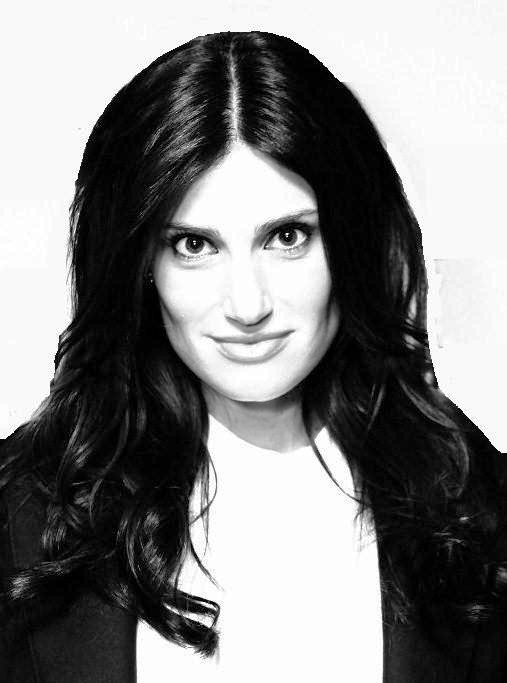This black-and-white photograph features a woman in her early to mid-thirties, captured with a very bright and highlighted effect. She has long dark hair, parted in the middle and styled in layers with a nice wave that reaches just below her shoulders. Her dark eyes, enhanced with makeup, gaze intensely and happily straight into the camera, complemented by a subtle yet visible smile. The lighting casts a shadow on her neck while making her face and upper chest area exceptionally bright. This strong lighting creates an almost digitally altered look, particularly noticeable around the edges of her hair against the completely white, featureless background. She wears a white inner top paired with a dark jacket or blazer.